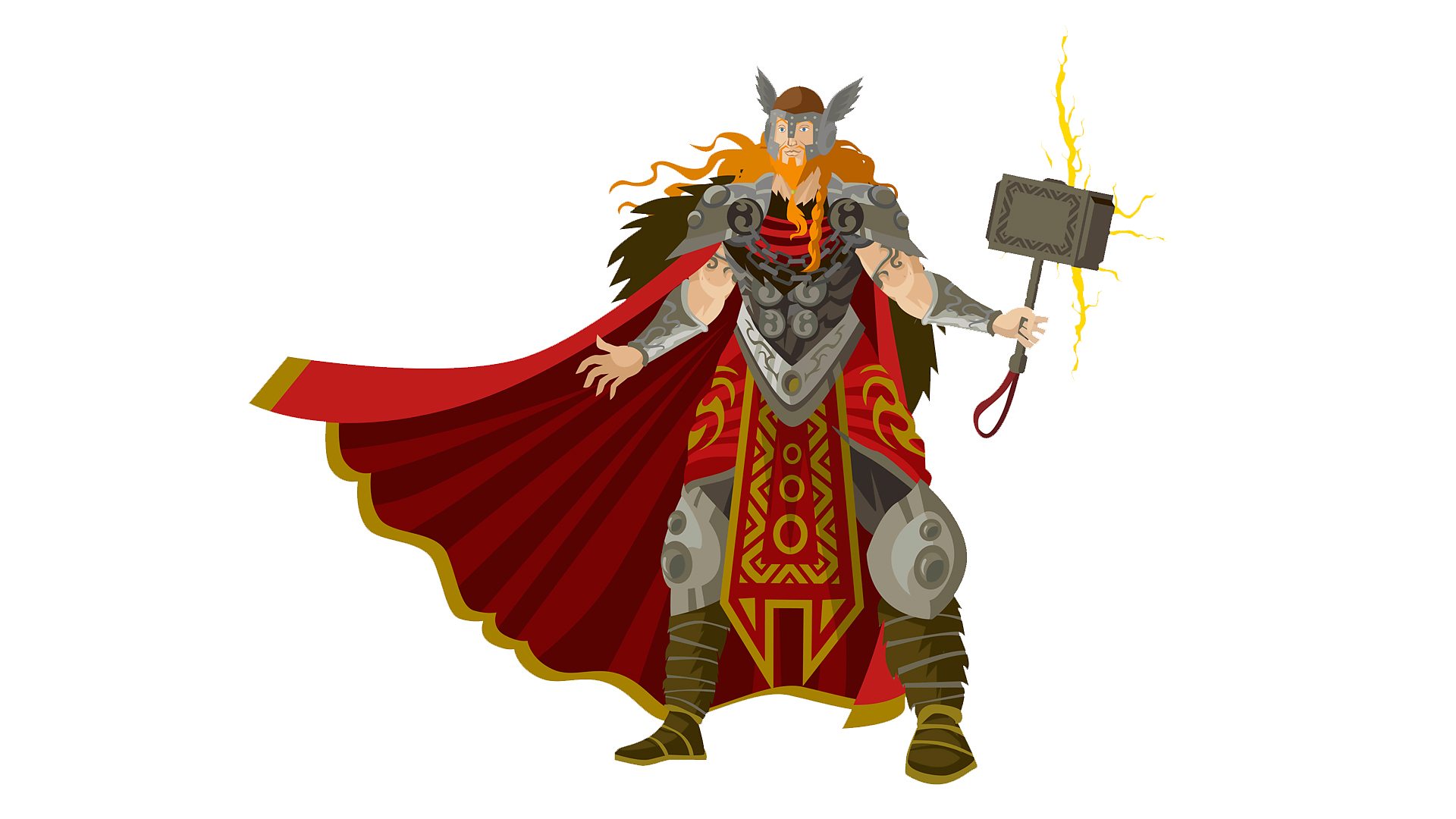This image features Thor, the mighty Norse god of thunder, depicted in detailed attire and stance. He commands attention with his long, flowing reddish-orange hair and a striking silver helmet adorned with ornate silver wings. Thor is clad in a distinctive brown top, revealing muscular arms, and his protective armor which does not fully cover his limbs. His forearms are shielded by robust metal wrist braces, while hefty, metallic shoulder plates enhance his imposing presence. The main body armor is designed like a sleeveless tank top, predominantly red in the middle, with a gray section beneath it, framed by a lighter gray border that cinches around his waist. From his waist down, Thor sports a red wraparound garment, accented in the center by a striking yellow and red vertical strip. His knee armor mirrors the design of his shoulder plates, complemented by durable brown boots. Draped across his back is a majestic red cape, edged with a bright yellow border. Grasped firmly in his hand is Mjolnir, his legendary hammer, characterized by its short handle and large, rectangular block-head, fashioned from what appears to be two merged squares. Electrifying bolts of lightning emanate from Mjolnir, capturing the awe-inspiring power Thor wields. The image zeroes in solely on Thor, devoid of any background distractions, highlighting his mythic and heroic essence.